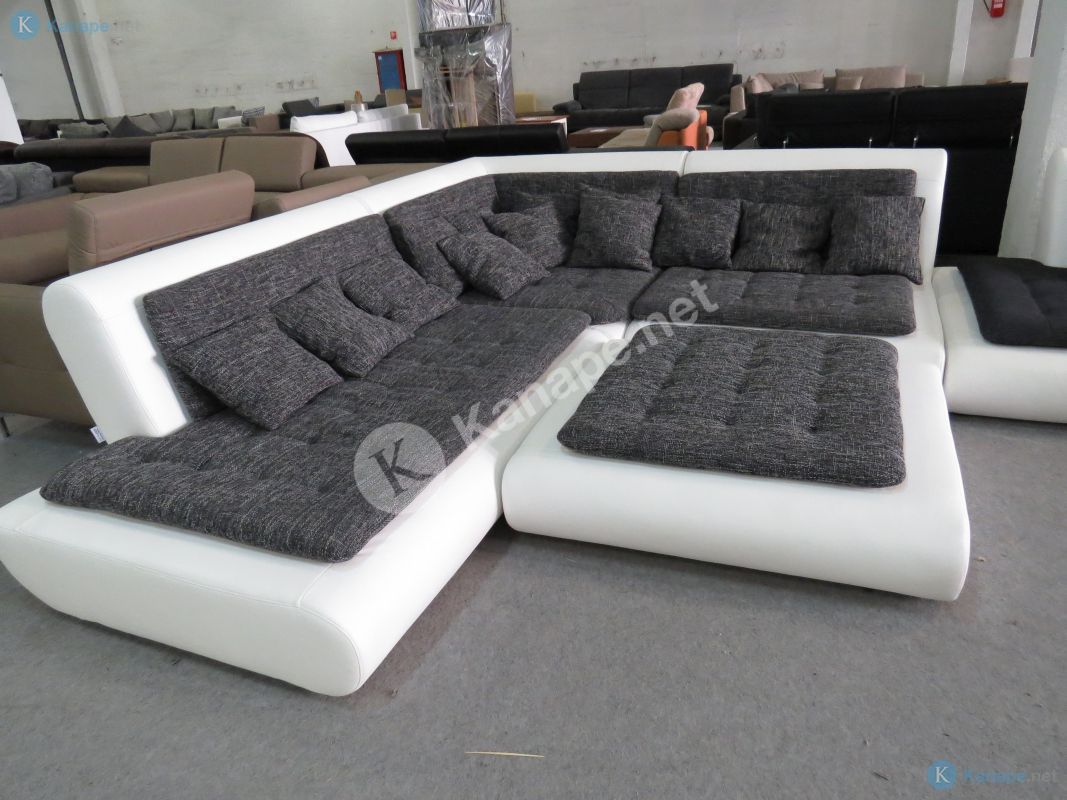This image showcases a modern sectional sofa situated within a furniture showroom, possibly a factory setting. The space is filled with various chairs and sofas against a backdrop of a worn, white wall. The main focus is the low-to-the-ground, L-shaped sectional which features a bright white fabric exterior. The seating area is accentuated by dark gray pads on the seats and backs, with a line of matching gray throw pillows enhancing comfort and style. Additionally, a similarly designed ottoman, mirroring the color scheme and pattern of the sectional, sits directly in front. A noteworthy detail is a diagonal logo across the front of the couch, displaying a "K" at the center beside the text "Canapé.net," adding a touch of branded modernism to the piece.